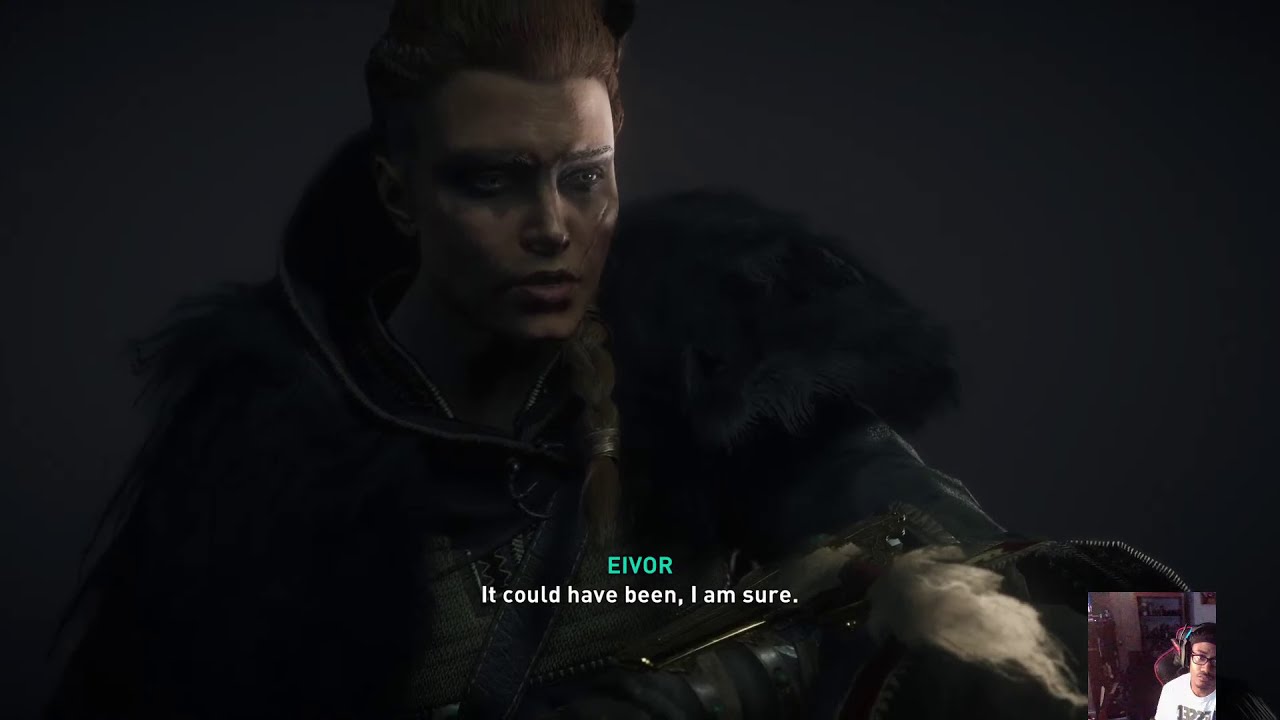The screenshot depicts a moment in a 3D multiplayer video game featuring a dark, fantasy setting. Dominating the screen is a medieval character, dressed in a black fur-collared leather jacket and adorned with battle scars. This character, identified by the green text "EVOR" at the top of the subtitles, has brown hair tied back with a brass ring and appears to be looking slightly concerned as they slide to the right, partially lit with shadows casting across their face. Below the character’s name, white subtitles read, "it could have been, I am sure."

In the bottom right corner of the screen, there's a smaller inset showing a young man live streaming his gameplay. He is wearing black glasses, a white shirt with indistinct black text, and a headset featuring a green band on the top. His dimly lit room has a reddish glow, a cabinet on the left, and a door in the background, adding to the immersive and atmospheric ambiance of the scene.